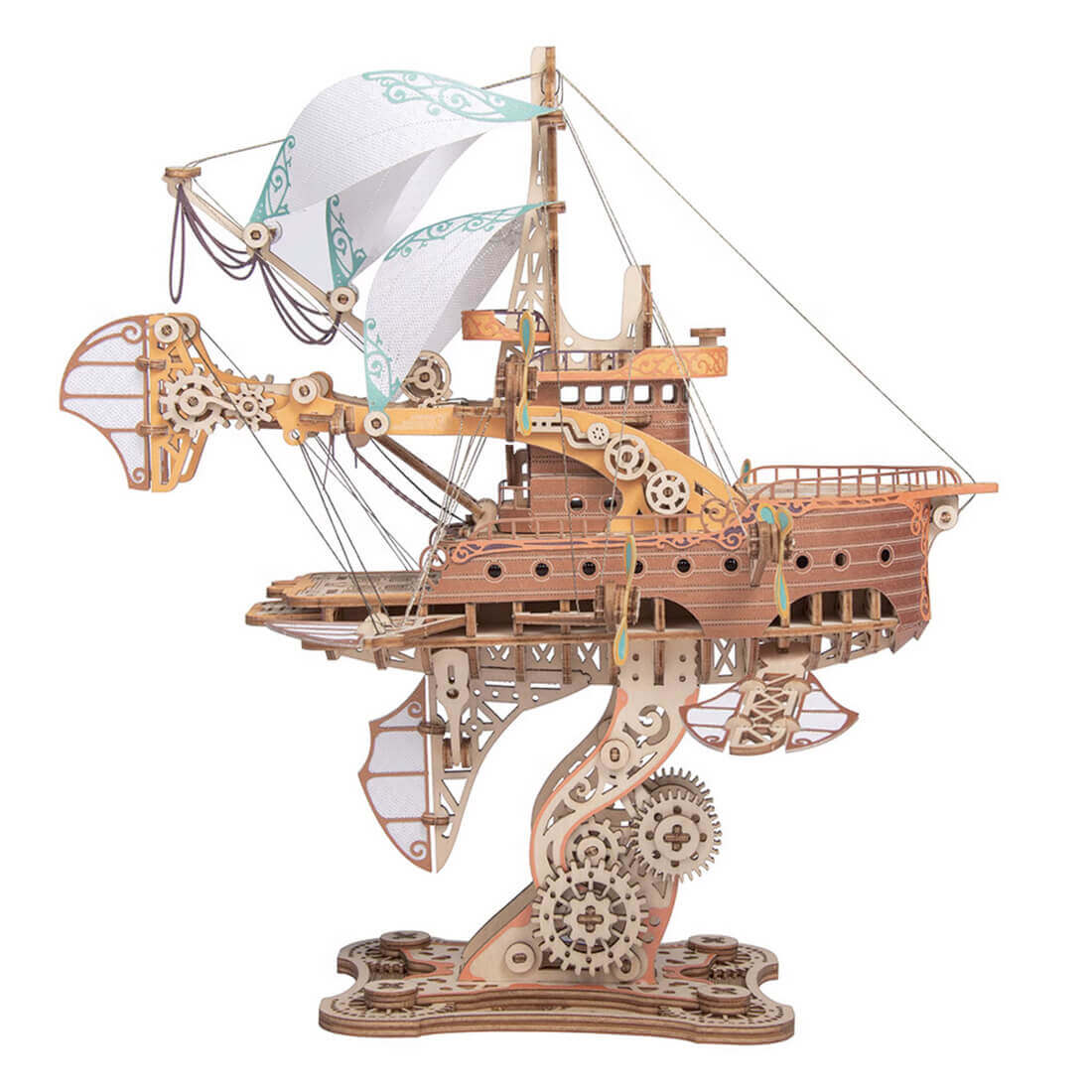This image features an intricate and elaborate wooden steampunk-style pirate ship that appears to be either flying or floating. The ship is positioned on a complex base that resembles a clock mechanism, adorned with numerous gears visible throughout the structure. The base, along with the gears extending to the sides and front of the ship, suggests a mechanical nature, combining elements of both nautical and timepiece designs. The ship itself boasts three white paper sails with blue and green designs, adding to its decorative charm. An elaborate cabin sits in the center, and there is a mast towards the back. The front and rear of the ship are equipped with wings, enhancing its fantastical aesthetic. The overall color palette includes shades of brown, orange, beige, white, and mint green, giving it a warm yet whimsical appearance. The background is stark white, highlighting the detailed craftsmanship and sophisticated construction of this intricate wooden masterpiece.